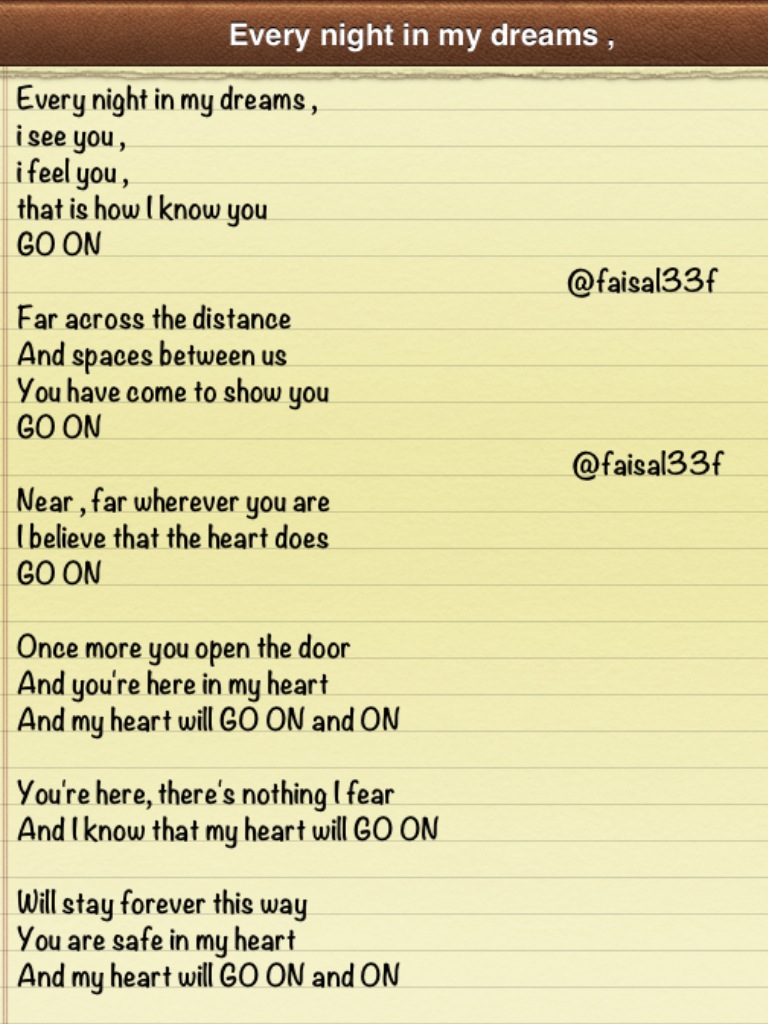The image appears to be a screenshot from an old Notepad app, featuring a skeuomorphic design with torn paper below a leather-bound heading. At the top, a brown title bar displays the text "Every Night in My Dreams" in white. Beneath this heading, a piece of yellow-lined paper contains the handwritten lyrics to Celine Dion's song "My Heart Will Go On." The text begins with "Every Night in My Dreams, I see you, I feel you, that is how I know you go on. Far across the distance and spaces between us, you have come to show you go on." It continues with familiar lines such as "Near, far, wherever you are, I believe that the heart does go on," and "Once more, you open the door, and you're here in my heart, and my heart will go on and on." The passage concludes with "You're here, there's nothing I fear, and I know that my heart will go on. We'll stay forever this way. You are safe in my heart, and my heart will go on and on." Notably, user handles such as "Faisal33F" are inscribed on the right side of the Notepad, indicating potential authorship or annotation.